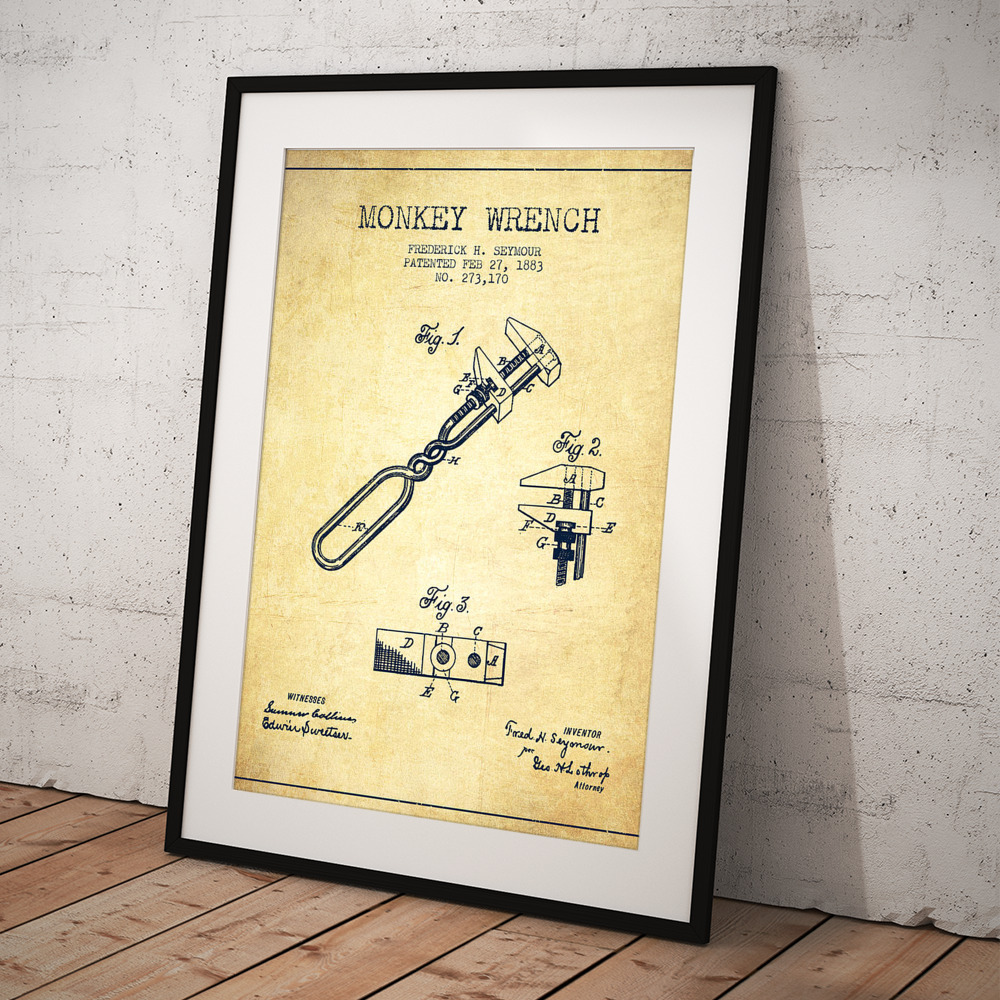This image is a framed photograph of an old patent for a monkey wrench, leaning against a white brick wall with tan wooden flooring. The black frame features a white border, showcasing a tan canvas that presents intricately detailed illustrations and descriptions. The top of the canvas is labeled "Monkey Wrench," followed by the inventor's name, Frederick H. Seymour, and patent details: February 27, 1883, Patent No. 273,170.

The central focus of the canvas is a series of technical sketches. Figure 1 is the largest, depicting the full monkey wrench with various components labeled A through I, including the jaws and screws that adjust the wrench's grip. Figure 2 offers a side view of the jaws, illustrating how the distance between them can be adjusted. Figure 3 provides a detailed top view of additional mechanical parts. Annotations highlight clamping mechanisms, screwing mechanisms, and other essential components that facilitate the wrench's operation.

The bottom of the canvas includes signatures for witnesses, the inventor, and the attorney, emphasizing the official nature of the document. This piece not only showcases the mechanical ingenuity of the 19th century but also serves as a historical artifact documenting the formal patent process.